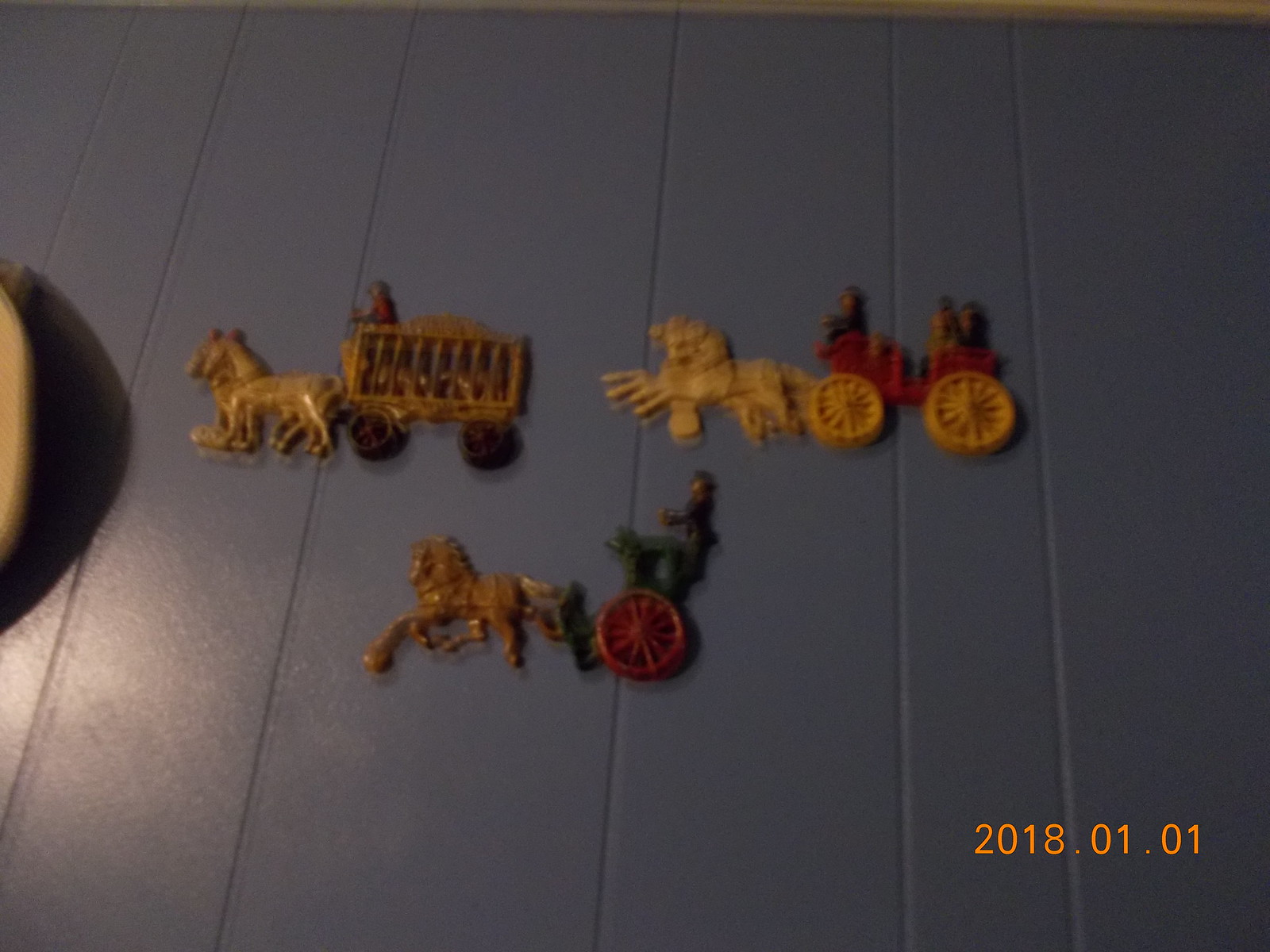The photograph showcases a dark blue wooden wall adorned with three detailed, slightly three-dimensional horse-drawn carriage decorations, which appear somewhat blurry and underexposed. On the upper left, there is a caged carriage reminiscent of old carnival wagons, pulled by two cream-colored horses, with a man in a red shirt, gray hat, and blue pants sitting on top. This carriage has large black cast iron wheels. To the right, a scene features two white horses galloping, pulling a red carriage with tan wheels, carrying three individuals; one man in black, seated at the front, appears to be driving. Below these two, there's a single bronze horse in motion, pulling a small green carriage with a red wheel, driven by a man in dark blue standing on a platform. Another object casting a shadow can be seen to the photo’s left edge but is partially cut off and indistinct. The image has a date stamp of January 1, 2018, in the bottom right corner.